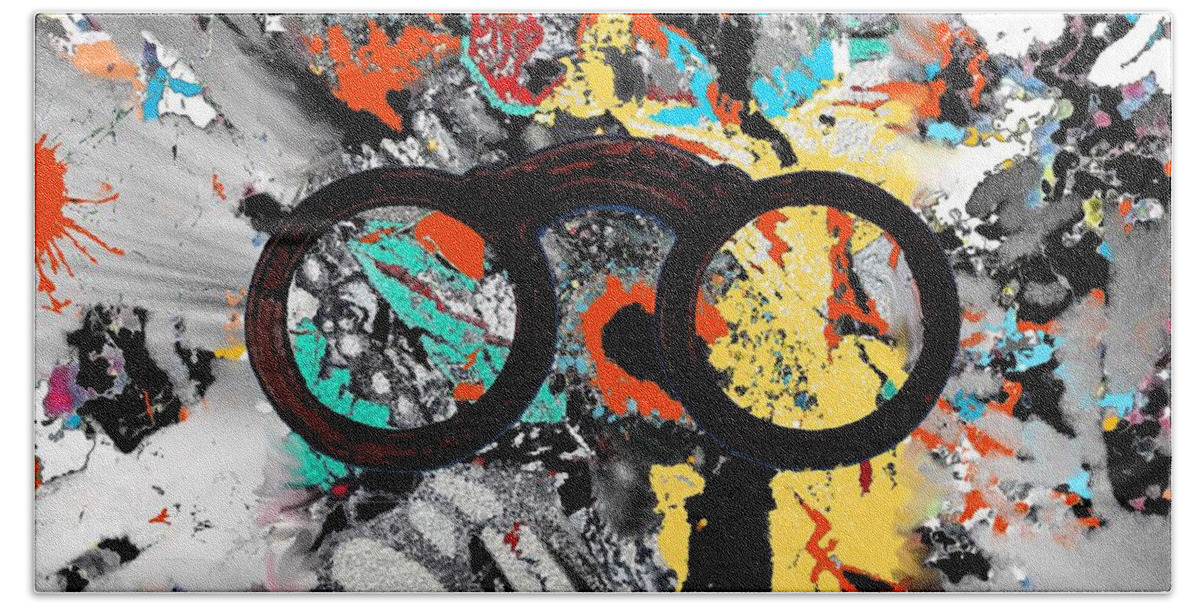This image showcases an abstract rectangular artwork, characterized by an explosion of vibrant colors set against a predominantly gray background. Central to the piece are two black circles connected at the top by a small bridge, resembling either spectacles or a rudimentary bicycle. The dynamic background features a cacophony of paint splatters and designs with colors including red, yellow, blue, light blue, teal, white, black, purple, orange, and pink. The abstract design extends to all four borders of the artwork, suggesting a large and immersive piece.